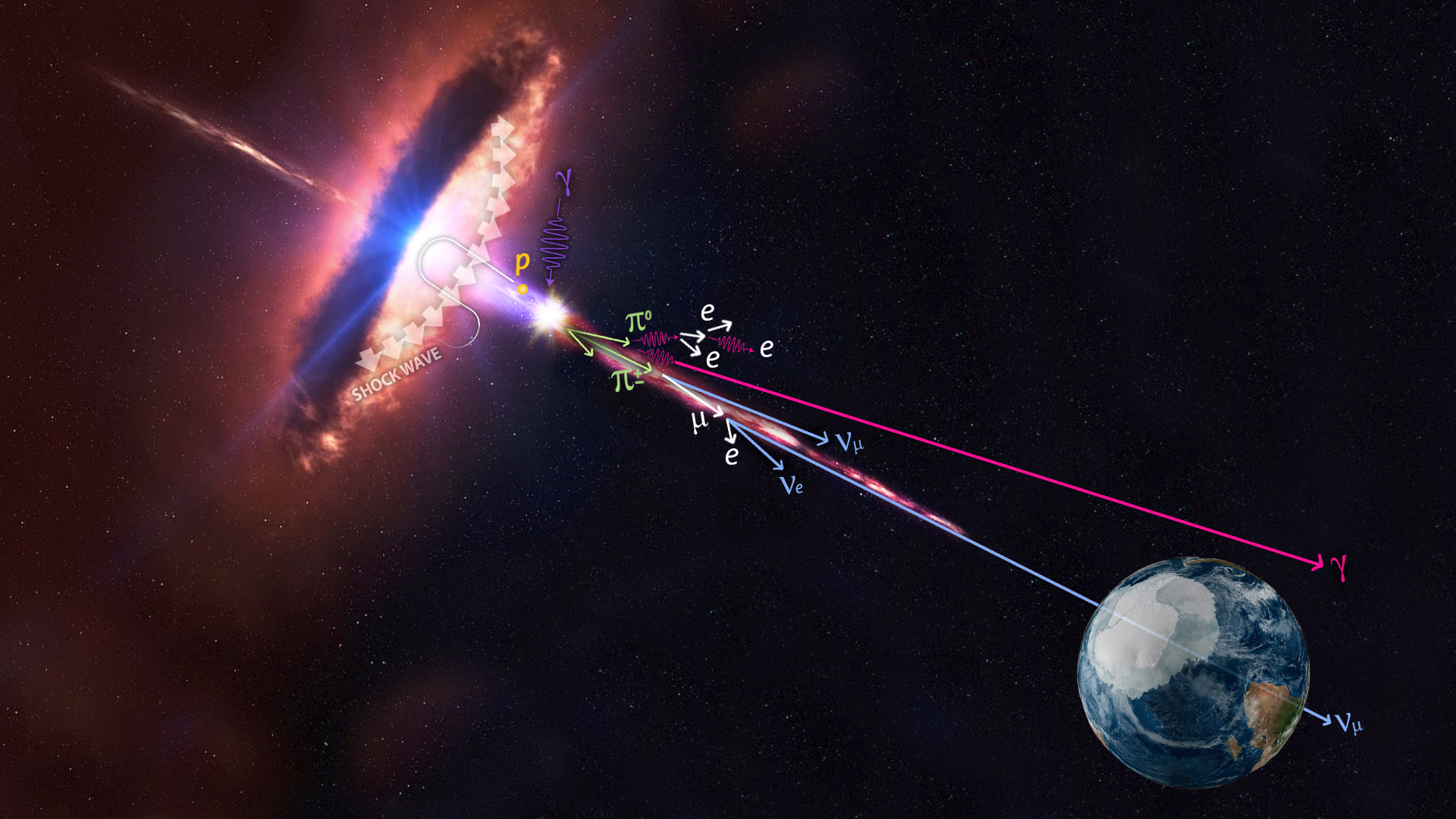This image showcases an Earth-like planet in the lower right corner set against a black background resembling deep space. In the upper left, there is a prominent, bright explosion-like circle emitting a multicolored glow, with blue, white, and orange hues, creating a vivid shockwave effect. The circle is encircled by a large glowing ring, accompanied by a wavy white line at its base labeled "shockwave."

From this area, numerous multicolored beams and arrows radiate towards the planet. These beams and arrows, adorned with a variety of mathematical notations, exhibit a range of colors, suggesting complex physical or dynamical processes. Among these notations, green arrows are marked with different forms of the symbol π (pi), including one labeled "π₀" and another with an illegible subscript at this resolution. Alongside these, magenta lines, including one very long line leading to a Greek character resembling a capital Y (possibly a Psi or another similar letter), indicate additional mathematical variables or vectors.

Furthermore, the image includes various lowercase e's and Greek letters such as mu (μ) dispersed among the arrows, some of which are white and others blue. Three significant blue lines, one notably long and cutting through the planet, are labeled with 'V' and subscripts, indicating velocity vectors or similar quantities. The presence of a yellow P on a single point adds to the array of symbols within this visual explanation.

Overall, this complex and detailed diagram seems to illustrate a scientific model or phenomenon involving shockwaves, mathematical physics, and potentially astroengineering or space phenomena.